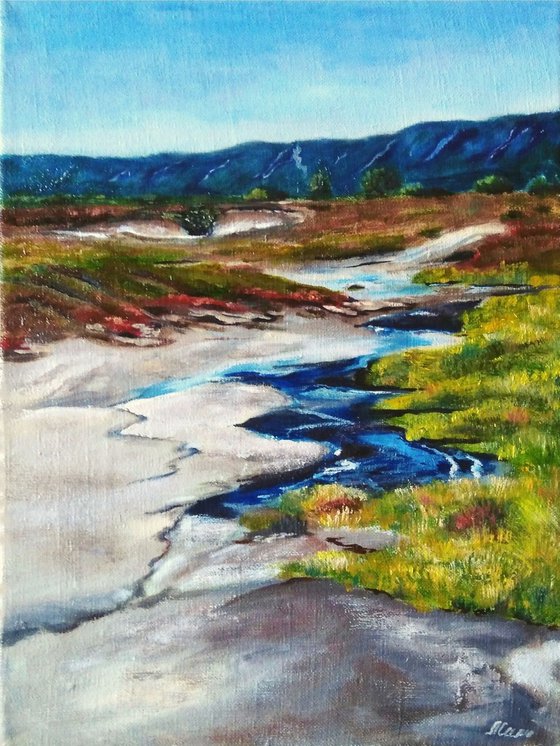The painting, which appears to be in oil on canvas, portrays a vivid and serene nature landscape in portrait orientation. Dominating the scene is a meandering river, winding vertically through the canvas with textured blue and gray hues that capture the flowing water. On the right bank, lush green grass and flourishing flora contrast with the river. The left bank features stark white patches of what seems to be solid salt or beach areas with grass and dirt patches and a small fallen tree limb crossing over the stream. As the river extends into the horizon, it is flanked by a diverse landscape; towards the middle ground, greenery transitions to dirt paths leading up to a distant, dark blue mountain range. The sky above is a light blue interspersed with frail, patchy white clouds, adding to the tranquil yet dynamic composition. Notably, the artist's signature is found in the lower right corner, although it is somewhat obscured and unclear, possibly reading as S. Classen or S. Casey. This detailed depiction brings to life the Kamchatka landscape within the crater of a volcano, capturing the natural beauty and varied textures of this striking environment.